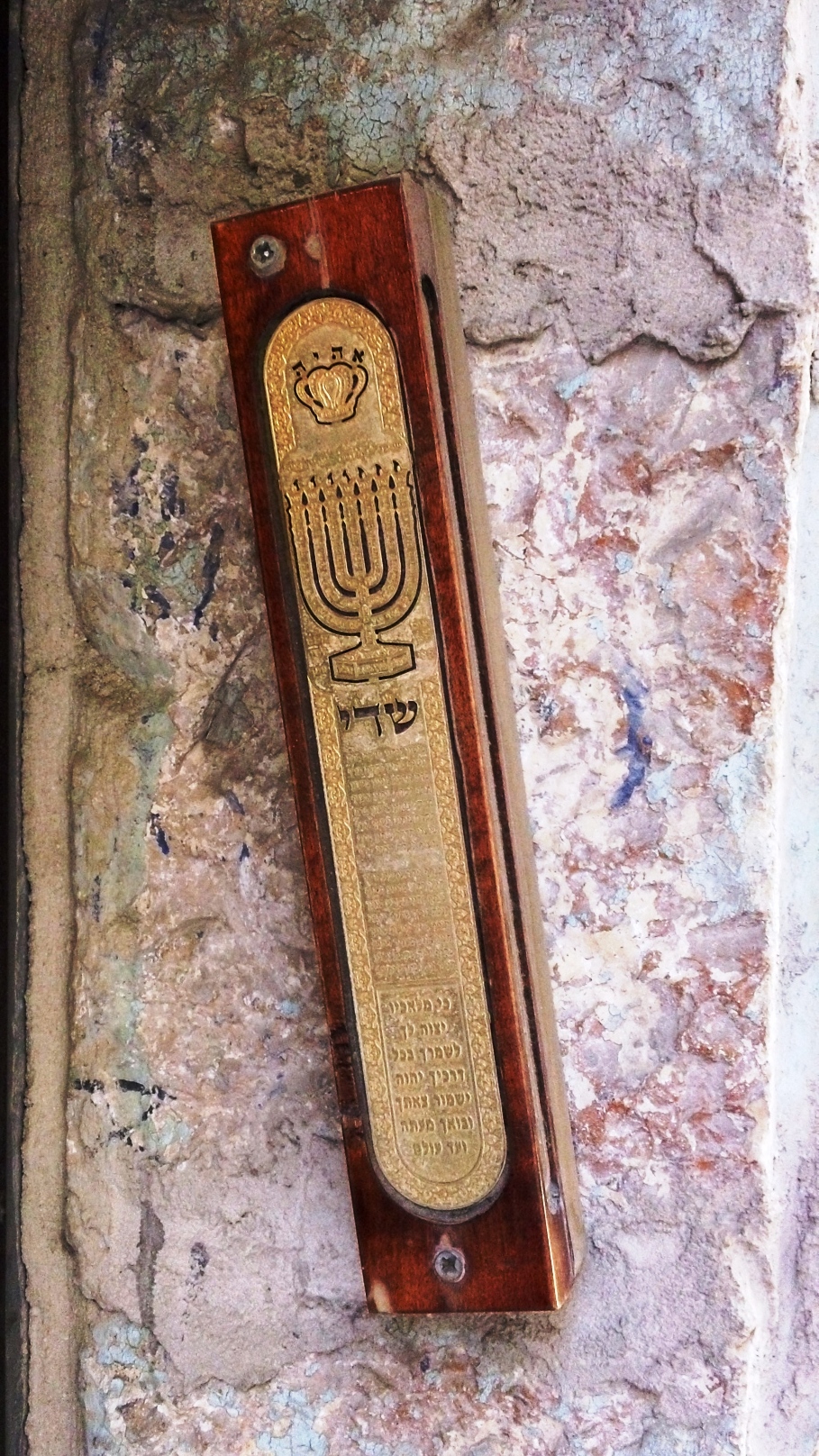The image features a mezuzah, traditionally affixed at an angle to a door or wall, that is shown here on a faded stone or brick surface with muted colors of tan, green, and faded red. The mezuzah itself is made of brown wood with a central gold section. The gold part features an engraving of a menorah with seven candles, and above it, a crown-like shape. The photograph, seemingly taken during daylight, captures the mezuzah against a backdrop of a white-brownish wall speckled with blue, white, and green hues. The overall setting hints at a residential building, contributing to the detailed and textured ambiance.